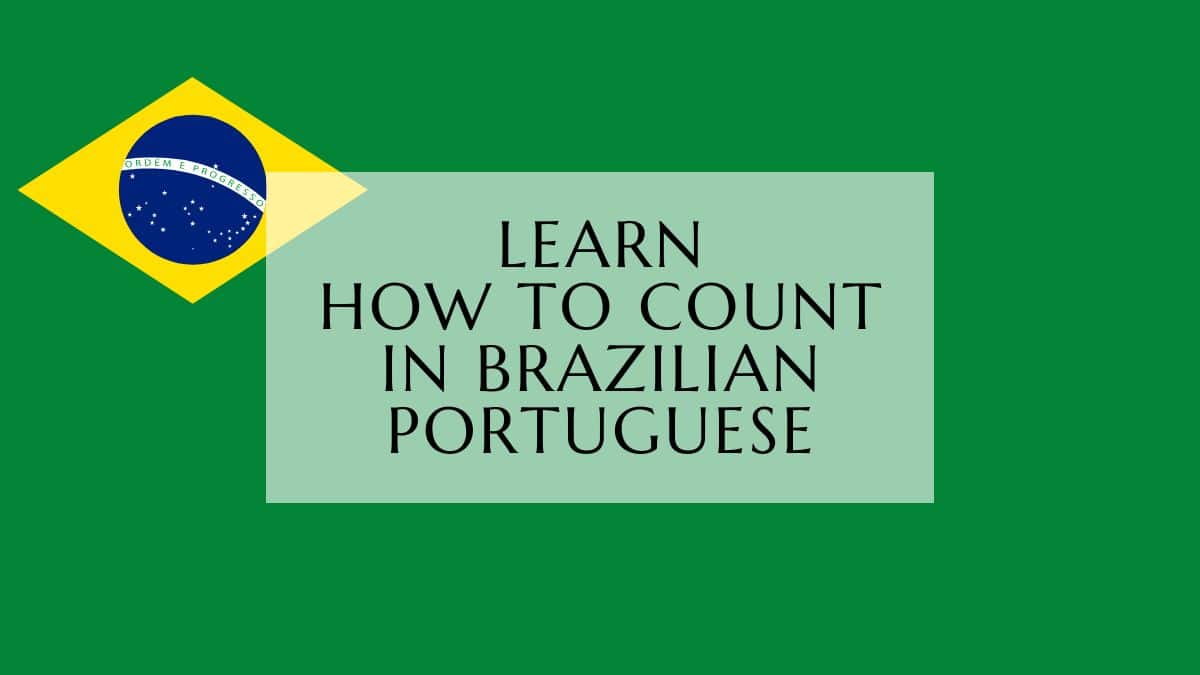The image features a green gradient background, which transitions from a light shade at the bottom to a darker shade at the top. Positioned towards the left side of the image is a yellow diamond, oriented horizontally with its longest side. Within the diamond, there is a blue depiction of the Earth, showcasing a starry sky along with the phrase "Ordem e Progresso" in white uppercase letters circling the globe. To the right of the yellow diamond, there is a green rectangle containing a bold message in black uppercase letters that reads: "LEARN HOW TO COUNT IN BRAZILIAN PORTUGUESE."